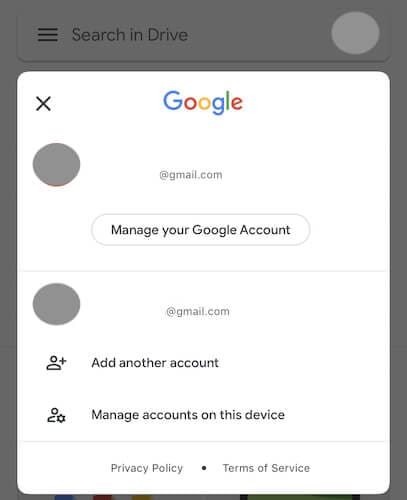A Google account management pop-up window overlays a screen with a "Search in Drive" feature. Visible at the top of the underlying screen are three horizontally stacked black lines and a white circle icon on the right, all covered by a semi-transparent gray overlay. 

In the center of the pop-up window, there is a vertically elongated white rectangle displaying "Google" and an associated email address ending in "@gmail.com". A black 'X' is positioned at the top-right corner. Below the email address, on the left side, a grayed-out circle indicates the removal of the user's profile picture and Gmail name.

The pop-up also features a button labeled "Manage your Google account" in black text with a white background and a gray outline. A horizontal gray line separates this section from another grayed-out circle and anonymized Gmail name below it.

Further options include "Add another account" and "Manage accounts on this device", separated by a horizontal line. At the bottom, links to the Privacy Policy and Terms of Service appear in gray text with a black dot separator. The overall color scheme uses a mix of black and gray fonts, emphasizing the privacy and account management functionalities, while omitting personal details for confidentiality.